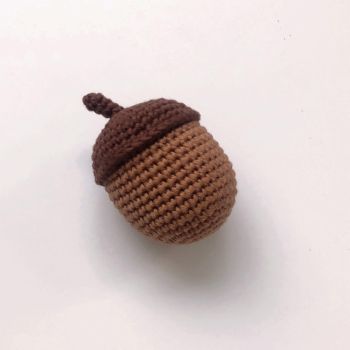This image showcases a meticulously crocheted acorn resting on a pale cream square-patterned background. The acorn features a rich dark brown cap (cupule) with a matching stem pointing northwest, while the rounded body of the acorn is a lighter brown, extending towards the southeast. The crochet work is fine and delicate, with the body displaying a small square pattern and the cap adorned with lined ridges. There is no accompanying text or website reference, and a subtle shadow beneath the acorn adds dimension to the composition.